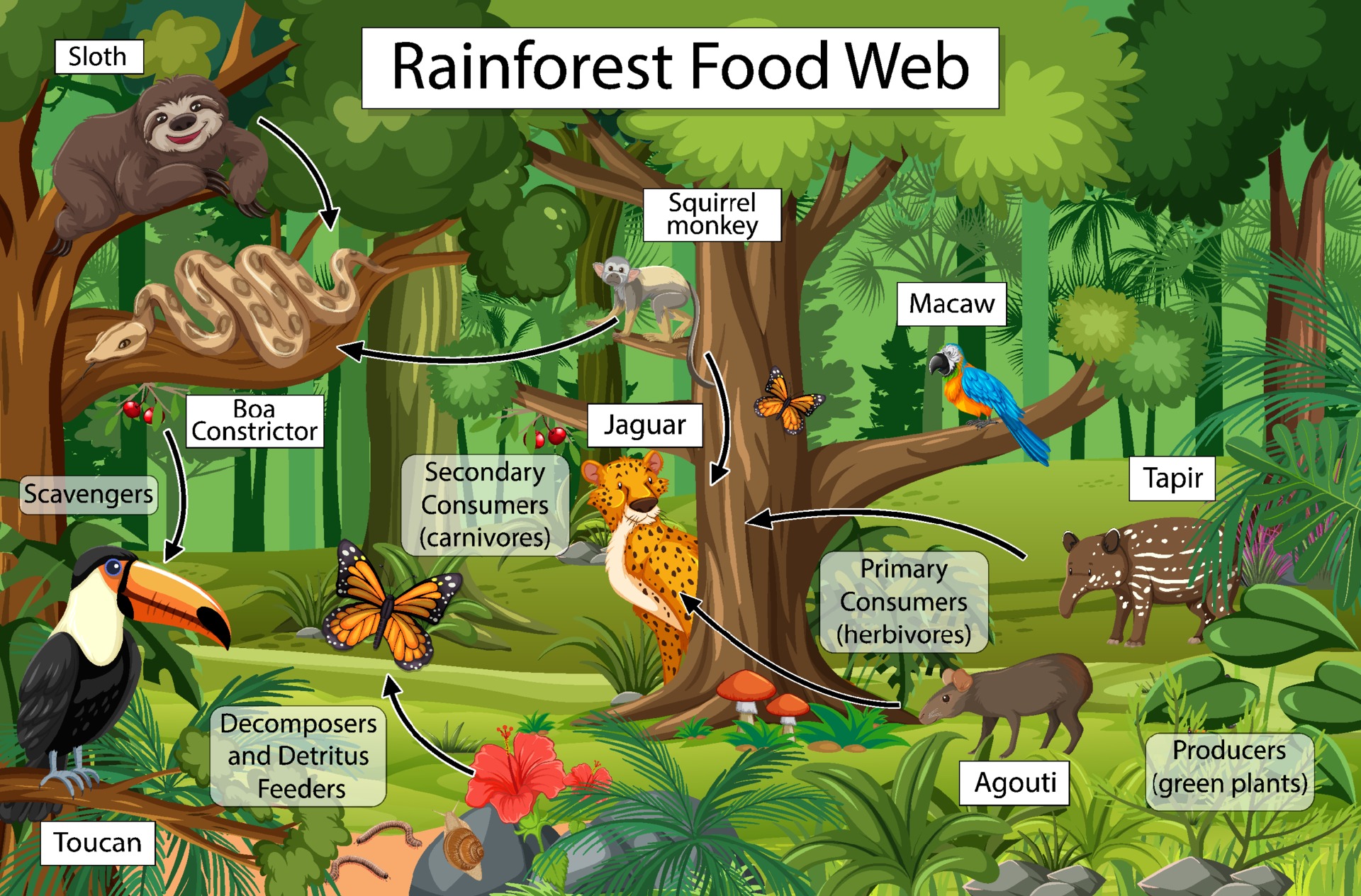This digital illustration, possibly from an educational textbook for young students, serves as a detailed depiction of the rainforest food web, complete with cartoon-like representations of various animals. The title "Rainforest Food Web" is prominently displayed at the top in black text within a white rectangle. Each animal within the lush, forested scene is clearly labeled with both its name and its role in the ecosystem. 

In the upper left, a sloth is dangling from a tree branch, labeled "sloth" with supplemental details indicating its classification. Below it, an arrow points to a resting boa constrictor, also situated on a tree branch. Another arrow links this boa to a nearby toucan, accompanied by a label denoting it as a scavenger. Additional arrows direct attention to decomposers and detritus feeders like snails, worms, and flowers on the ground.

On the right side, a colorful macaw with blue feathers and an orange chest tuft perches on a tree next to a squirrel monkey, both labeled accordingly. Further down, leaf clusters are identified as "producers, green plants," substantiating the food web's foundational layer. Close by, a tapir and an agouti are marked as primary consumers and herbivores.

Nearby, a monarch butterfly—or a similarly patterned insect—carries a label indicating it is a secondary consumer and a carnivore. Positioned prominently behind the central tree, a jaguar stands out with a label confirming it as a secondary consumer and carnivore. 

Arrows interconnect these various animals, illustrating the complex network of predation and consumption integral to the rainforest ecosystem, with each element clearly defined to aid understanding.